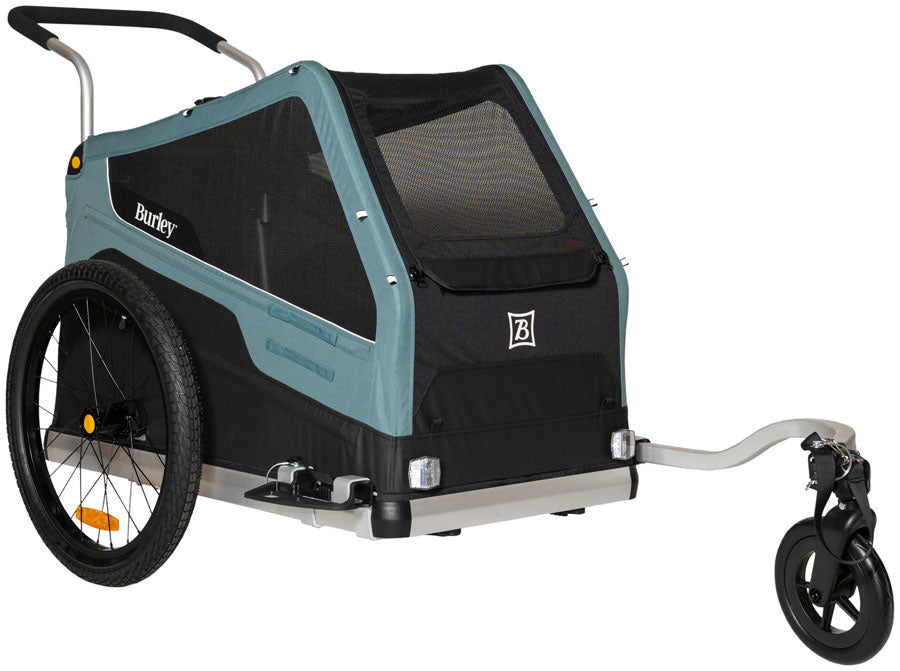The image depicts a wheeled carrier, identifiable as a Burley, primarily used for transporting children. The carrier has a distinctive setup, featuring a robust, large black wheel on the back that resembles those found on wheelchairs, along with a smaller front wheel supported by a metal rod extending from the right side of the carrier, curving towards the center to maintain balance. The front of the carrier prominently displays a "B" logo, and the name "Burley" is visibly printed on its black nylon sides in white letters. The covering of the carrier includes netting on the sides and a Velcro-sealed front area, providing visibility and access to the interior space, which is intended to accommodate a child. Handles are attached to the back of the carrier for manual pushing or pulling. The overall design includes both functional and safety features, making it versatile for use as a child transport unit that can be either pushed by hand or attached to a bicycle.